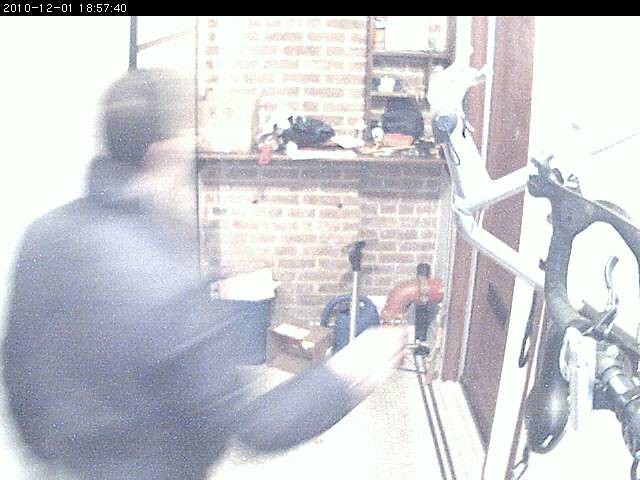The image depicts a grainy, security camera-style photo captured on December 1, 2010, at 18:57:40, as indicated by the timestamp on the top left corner. The scene takes place in a room with a stone or brick wall in the background, where shelves hold various items. A man with black hair, dressed in a black jacket, is slightly blurred due to movement, suggesting he is in the middle of an action. Positioned from behind, his face is not visible, but he appears to be reaching for something with one hand extended forward. To his right, there is a metal contraption, likely a piece of exercise equipment, situated in front of a brown door. The floor is cluttered with various objects, including a garbage can, a vacuum cleaner, and a red pipe.